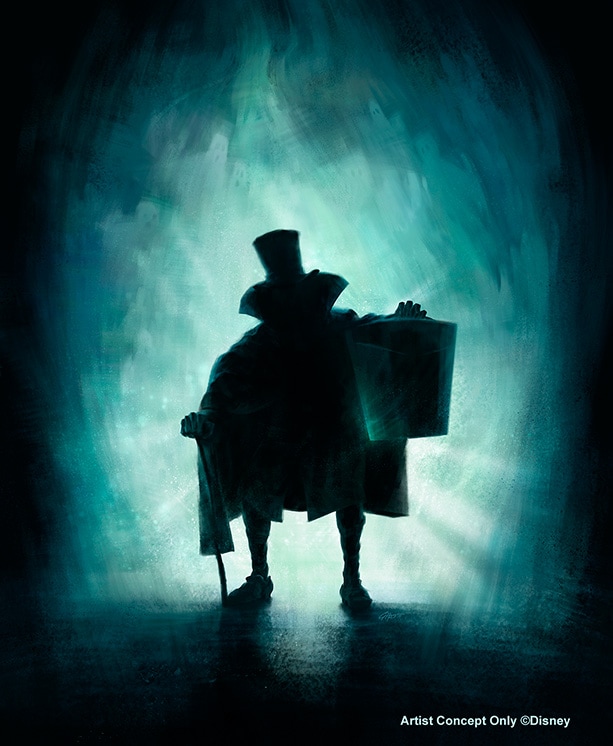This image, likely an advertisement for a Disney movie, is labeled "Artist Concept Only, Copyright Disney" in light green text at the bottom right. The vividly rendered scene, either hand-painted or computer-generated, features an eerie, shadowy character set against an ombre background that transitions from black at the edges to shades of blue and green toward the center.

The central figure, backlit to reveal only a dark silhouette, wears a top hat and carries a cane. His attire includes loose leggings and crude shoes, while in his left arm, he holds up a round or cylindrical object towards the viewer. The striking lighting from behind obscures any facial features, adding to the mystery. Surrounding him, the whitish-green illumination faintly reveals spectral green and white markings resembling ghostly eyes and mouths. The overall atmosphere is dark and somewhat creepy, evocative of ghostly aura emanating from the character.